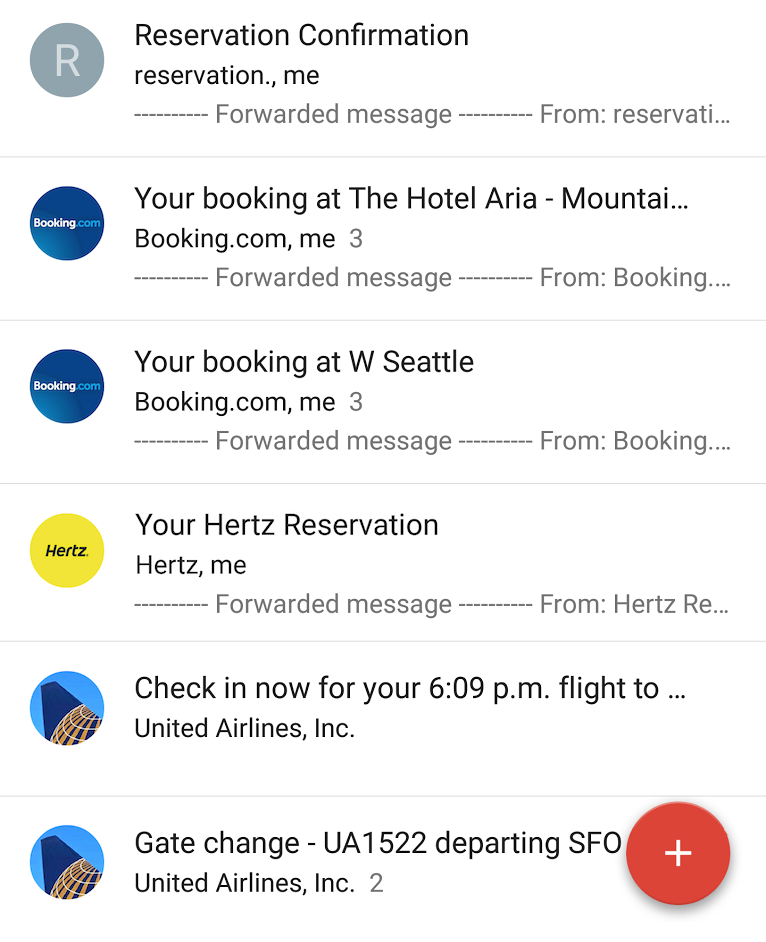Here's a cleaned-up and detailed caption for the image:

"A series of forwarded confirmation emails are displayed, pertaining to various reservations and bookings. The first email confirms a reservation, simply stating 'reservation confirmation,' followed by a forwarded message. The next set of emails involve booking.com and detail bookings at two separate locations: Hotel Aria Mountain and West Seattle, with accompanying logo imagery featuring the booking.com blue logo. There is also a forwarded message regarding a car rental reservation from Hertz, showcasing their yellow logo with black lettering. Additionally, there is an email from United Airlines indicating a check-in notice for a flight scheduled to depart at 6:09 PM, followed by another email confirming a gate change for flight UA1522 departing from San Francisco (SFO) to an unspecified destination. The emails collectively capture a sequence of travel arrangements, exemplifying meticulous planning for an upcoming trip."